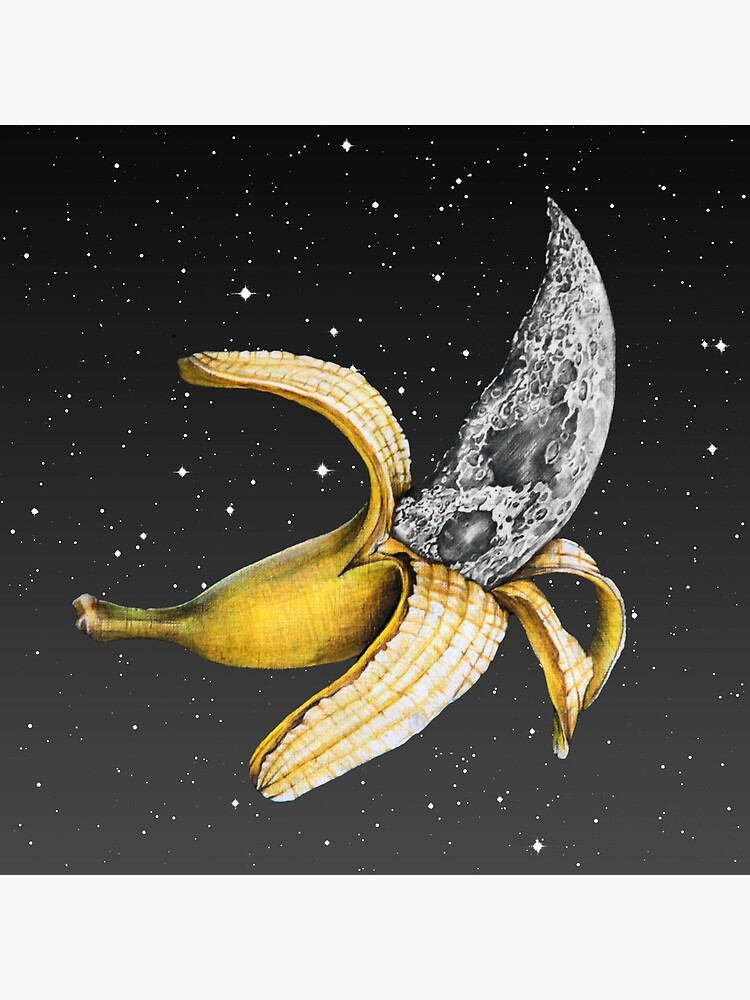In a beautifully detailed computer-generated artwork, a wide vertical rectangular image features a surreal scene set against a black outer space background, dotted with numerous white stars. At the heart of this illustration lies a partially peeled banana. Unconventionally, the banana is peeled from the bottom, with the yellow peel curling to the sides and upwards in a crescent moon shape. Intriguingly, the body of the banana is not yellow as one would expect, but instead reveals a surface resembling the moon—gray and craggy, dotted with white, circular bumps akin to craters. The banana curves from the bottom left to the upper right, emphasizing its lunar transformation. This whimsical depiction blends the familiar sight of a banana with celestial imagery, creating a rich and imaginative visual experience.